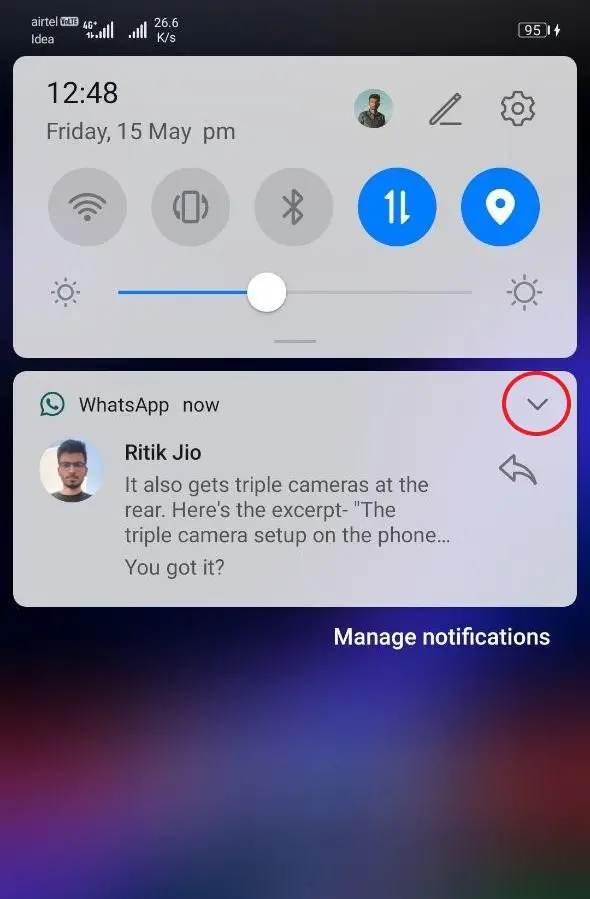The image displayed on a cell phone screen shows a detailed user interface with various elements. The status bar indicates a strong connection with 'Airtel' as the network provider and a battery level of 95%. In the upper part of the screen, there are two gray boxes. The first box shows the time as 12:48 PM on Friday, the 15th of May. 

Below the status bar, there is a profile image of a white male wearing glasses with a beard and mustache. Next to the profile image, there are two icons: one depicting a crayon and another for settings. 

Underneath, a set of larger-sized icons are visible, among which three are grayed out. The two active icons have blue backgrounds; the first one features the number one in two different orientations while the second one has a teardrop shape with a blue circle inside.

A slider control, used to adjust screen brightness, is positioned slightly to the left of the center, towards the dimmer side.

Further down, another gray box contains a notification from an app named 'What's Up Now'. The notification displays an icon of a character with a beard, glasses, and brown hair, identified as Rittik Geo. The message reads, "It also gets triple cameras at the rear. Here’s the excerpt: The triple camera setup on the phone. You got it?" This text is followed by a question mark and a drop-down menu, marked with a red circle and a left-pointing arrow.

At the bottom of this section, there is an option labeled 'Manage Notifications'. The background image of the screen features a beautiful, blended gradient of red, purple, and blue hues, giving it an aesthetically pleasing appearance.